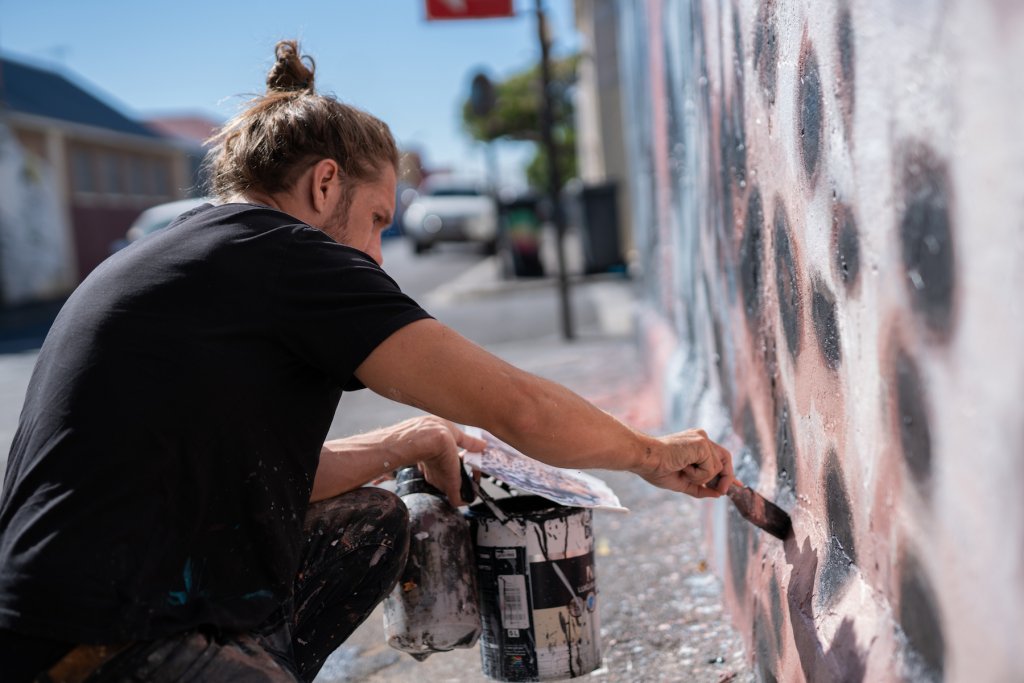The image depicts a young Caucasian male, likely in his late 20s or early 30s, with blonde, dirty hair styled in a topknot or man bun. He sports some stubble and a hint of a beard. Dressed in a black shirt and black pants, the man is actively engaged in painting a wall. In his right hand, he holds a paintbrush, while his left hand carries two cans of paint, one of which appears to be black.

The wall he is painting shows a blend of white, pink, and tiny black spots, giving it a polka-dotted appearance. The scene takes place outdoors during the daytime under a cloudy sky, likely in an urban residential area, possibly on the west coast of the United States given the architecture and overall setting.

The man is squatting slightly with his back and right arm prominently captured in the foreground, obscuring part of his face. Despite the clutter of paint on the floor, wall, and his clothes, the overall focus of the image is on him. The background is deliberately blurred, featuring a smattering of elements like a white car, a tree, a street sign, and some houses, but these details remain indistinct due to the photograph’s depth of field.